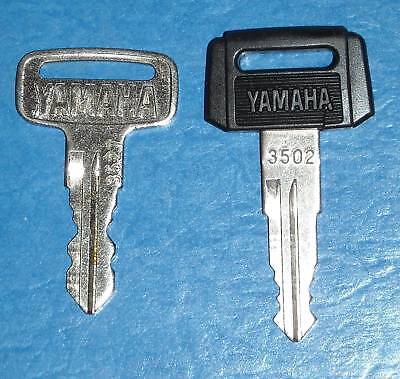The photograph features two vintage Yamaha keys lying on a slightly irregular seafoam blue or green surface, possibly a textured material like tarpaulin or a rubber mat. The key on the left is entirely silver with a long, wide loop on the head, and it bears the number 3527. This silver key exhibits a rough texture throughout. The key on the right has a black plastic head that is cracked, likely due to force applied to it, with the number 3502 stamped on it. Both keys have a distinct Yamaha branding, showcasing differences in design: the silver key is slightly wider, while the key with the black head is narrower. They are placed side by side in a close-up shot taken indoors with average quality, emphasizing their unique designs and condition.